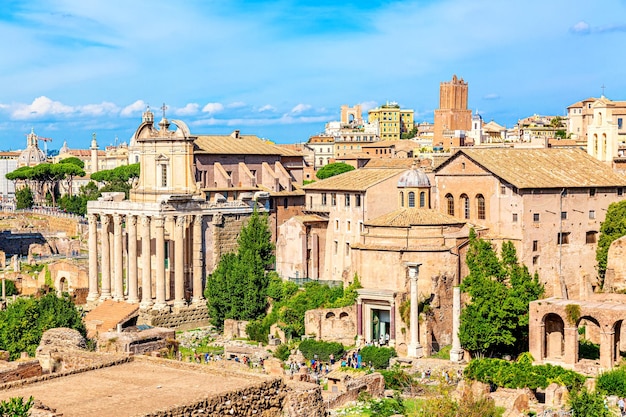The photo depicts an aerial view of a historical cityscape, possibly somewhere like Italy or Rome, showcasing a collection of tan stone buildings with architectural elegance. The buildings are tall, with some featuring several stories and adorned with columns and arch windows, particularly prominent on the left side where a structure with multiple tall pillars stands. 

On the left side, there's a notable flat rock platform with stairs leading up to it, appearing walkable and bordered by rugged rock edges. Adjacent to this platform, smaller, indistinguishable people can be seen milling about, their colorful attire—specks of blue, red, and white—providing a stark contrast to the muted stonework.

The scene is dotted with vibrant, green trees both around the buildings and in the background, enhancing the historical ambiance with natural beauty. Toward the right side, more buildings with fewer columns and some open archways are visible. In the distance, amidst the tan structures, there's a singular, slightly taller building with a darker brownish-red hue.

The sky overhead is a brilliant blue, transitioning from a deep azure at the top to lighter shades, punctuated by fluffy white clouds scattered horizontally and some wispy, misty ones higher up, adding depth and a dynamic atmosphere to the scene.